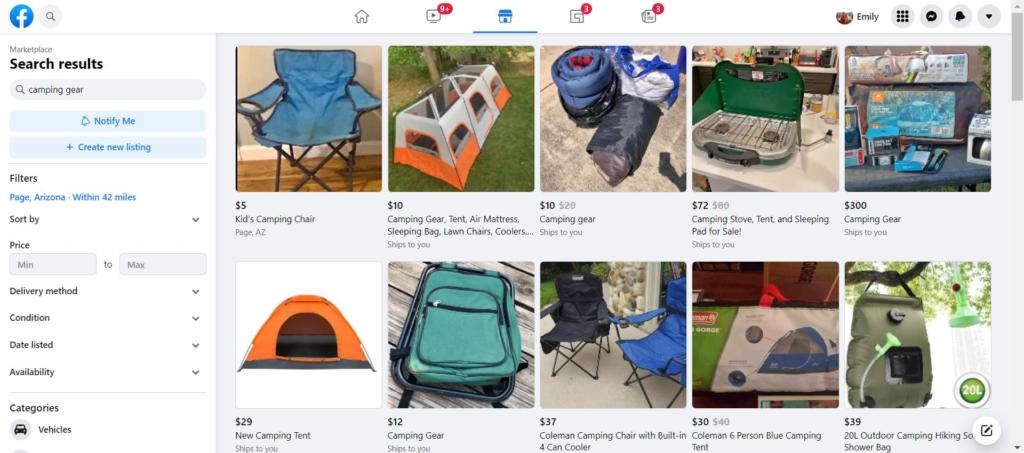This screenshot depicts a web page from Facebook Marketplace, showcasing a variety of camping gear available for sale. In the top-left corner, the familiar blue Facebook icon is visible, confirming the platform. The user, identified as Emily, is currently viewing the Marketplace section, which is noted in the vertical left-hand column labeled "Marketplace Search Results." Below this label, there is a search bar with the query "Camping Gear," followed by two blue buttons: "Notify Me" and "Create New Listing." Further filtering options below include: "Filters, Page, Arizona," "Within 42 miles," "Sort By," "Price," "Min to Max," "Delivery Method," "Condition," "Date Listed," "Availability," "Categories," and "Vehicles."

On the right-hand side of the page, a selection of Facebook Marketplace listings is displayed in a grid format consisting of two rows with five items each. Each listing features an image, a price, and a brief description. From left to right, the items listed include:

1. **$5 Kids Camping Chair**
2. **$10 Camping Gear**: Tent, Air Mattress, Sleeping Bag, Lawn Chairs, Coolers
3. **$10 Camping Gear**
4. **$72 Camping Stove**
5. **Tent and Sleeping Pad for Sale, $300 Camping Gear**
6. **$29 New Camping Tent**
7. **$12 Camping Gear**
8. **$37 Coleman Camping Chair with Built-in 4-Can Cooler**
9. **$30 Coleman 6-Person Blue Camping Tent**
10. **$39 20L Outdoor Camping Hiking Shower Bag**